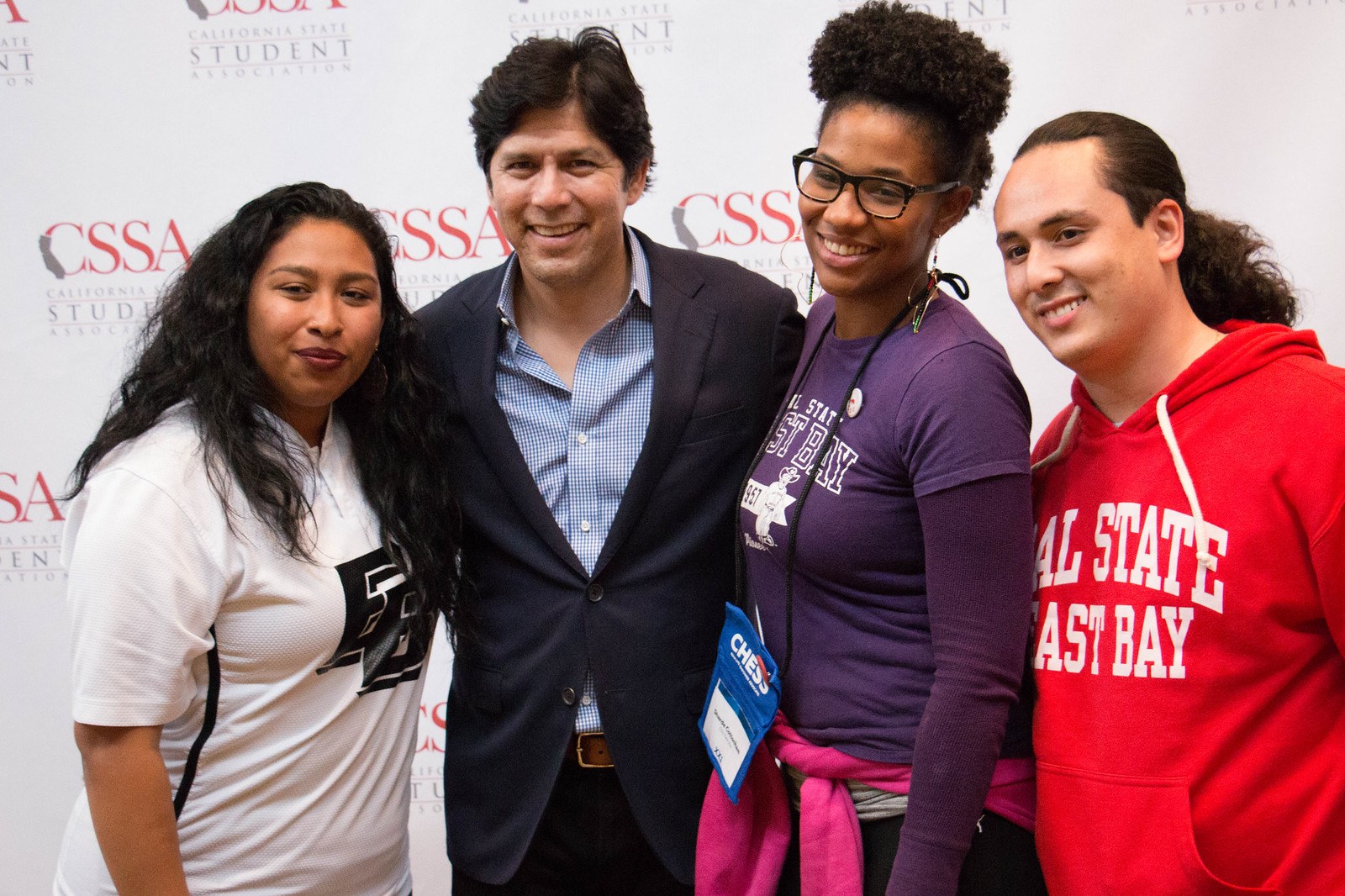This photograph features four individuals standing side-by-side, smiling warmly at the camera. They are posing in front of a backdrop prominently displaying the repeating initials "CSSA" and the full name "California State Student Association." The setting suggests an event, likely a conference or meeting organized by the California State Student Association, where various schools came together to discuss pertinent issues.

From left to right, the first person is a girl with long dark hair, wearing a white shirt adorned with black lettering. She looks cheerful and is smiling at the camera. Next to her stands a man in a navy sport coat and a blue and white checkered shirt. He has dark hair and extends his arms around the girl on his left and another woman to his right, indicating a friendly connection. The third person is a woman with dark hair styled in an updo, wearing glasses and a purple shirt. She sports a lanyard with a name tag and has a pink sweatshirt tied around her waist. The individual on the far right is a man with long dark hair tied back in a ponytail. He is also smiling and is dressed in a red hooded sweatshirt displaying the words "State" and "East Bay."

All four appear to be enjoying the moment, embodying the collaborative and positive spirit of the CSSA event.